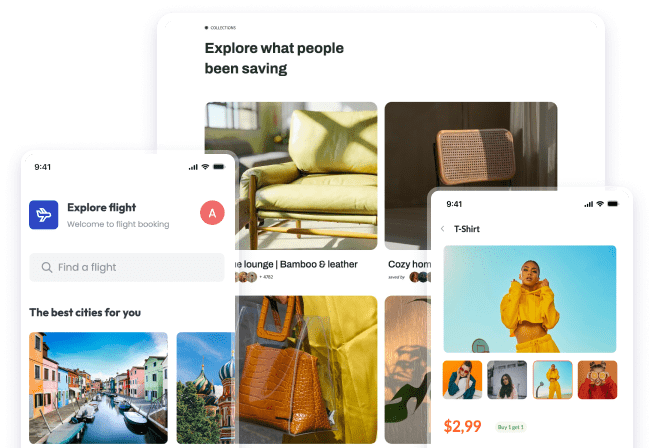This detailed caption describes a series of screenshots from what appears to be a travel and shopping platform, potentially Expedia:

"The image comprises multiple rectangular screenshots taken from an online platform, likely Expedia. The first screenshot features a promotional banner titled 'Explore Flight,' inviting users to book flights and discover top cities. The second screenshot showcases a section called 'Explore What People Have Been Saving,' displaying various saved items, including a couch and other personal goods. The final screenshot highlights a woman dressed in a vibrant yellow tracksuit, priced at $2.99. All screenshots are set against a clean, white background, enhancing the clarity and focus on the content displayed."